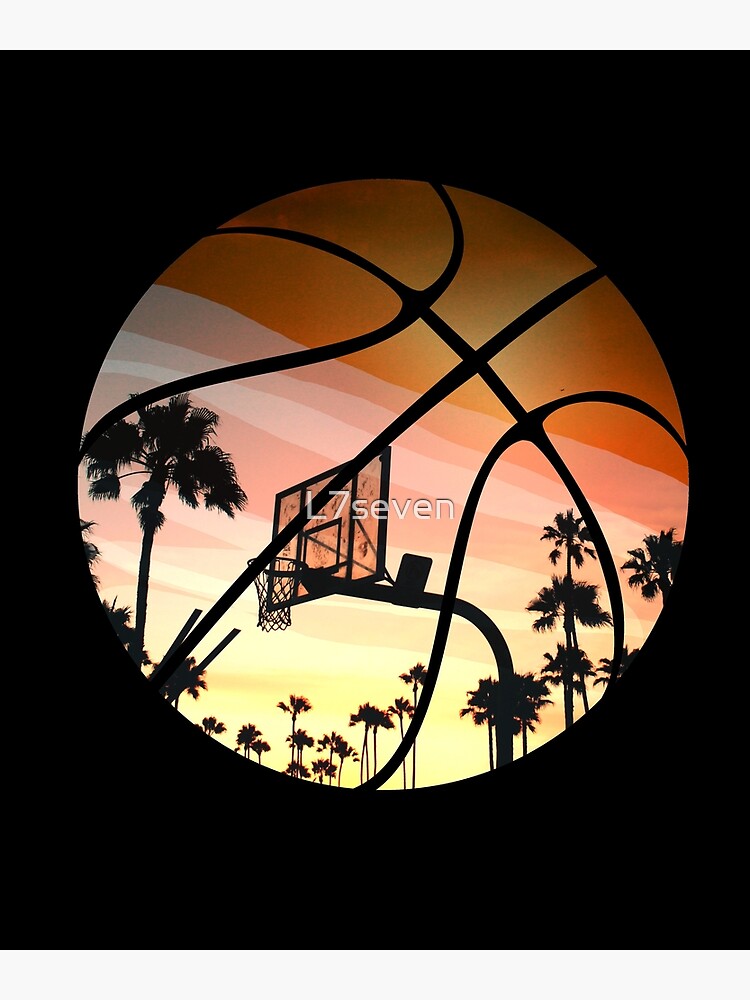The image is a distinctive piece of art featuring a stylized basketball set against a black background. The basketball is presented in a portrait orientation and appears slightly three-dimensional due to shading along its edges. The black seams on the basketball mimic the lines of a traditional basketball. In the top part, the ball is colored orange, transitioning into a vibrant sunset-like scene composed of various shades of pink and yellow as it descends toward the bottom.

Within the lower half of the basketball, there's an outdoor setting with silhouetted palm trees arrayed around the scene, giving it a California vibe. Centrally located is a basketball hoop and backboard, extending upward and enhancing the outdoor basketball ambiance. Superimposed onto this scene are the words “L7” and “7” in white, suggesting it could be a logo for an outdoor basketball initiative or event. This intricate blend of a natural sunset and a basketball theme makes the artwork striking and memorable.